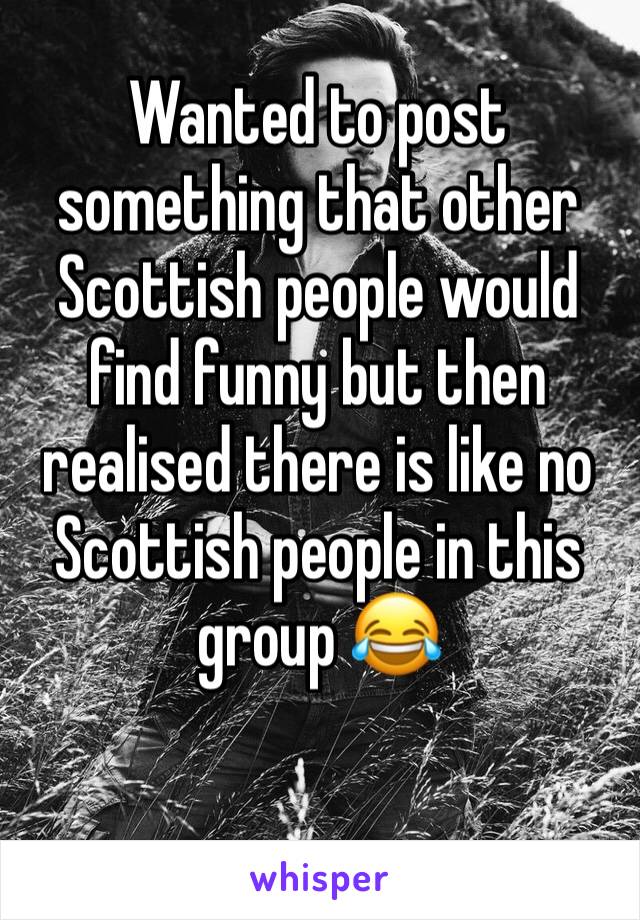This black and white meme image features a man standing in a field of tall grass, wearing a black button-down shirt open at the collar, with dark, slicked-back hair, and facial hair, possibly a mustache. Overlaid on the image is a humorous text in white font that reads, "Wanted to post something that other Scottish people would find funny, but then realized there is like no Scottish people in this group." The statement ends with a yellow laughing-crying emoji, showcasing a big grin with exposed teeth and blue tears on both sides. At the bottom of the picture, there is a small white banner with the word "whisper" in lowercase purple text. The overall composition merges rustic imagery with a modern humorous twist, intended to resonate with viewers familiar with niche online communities.